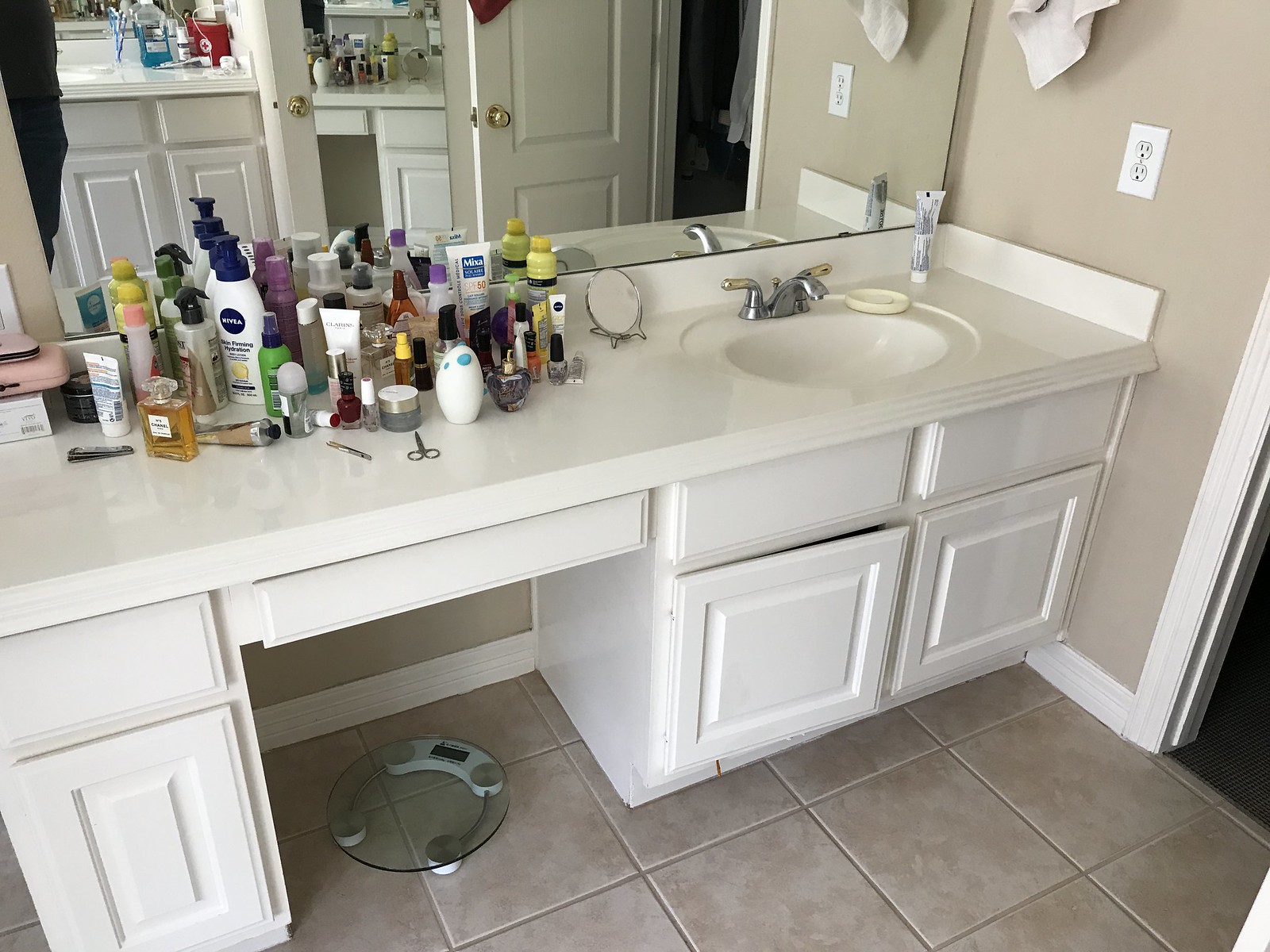The image captures a cluttered yet typical everyday bathroom scene. The floor is tiled in a warm, dark gray. The viewpoint is directed towards the bottom right corner of the bathroom, with a door entrance slightly visible there. Dominating the scene, a large mirror spans the length of an extended white countertop. 

To the far right of the countertop sits a single sink accompanied by a soap dispenser and toothpaste tube. Above the sink, a towel hangs and an electrical outlet is situated midway along the upper portion of the wall. The counter is cluttered with various personal items — from lotions and perfumes to everyday hygiene products like toothpaste, shampoos, and conditioners, making it difficult to itemize each one. 

Beneath the countertop are white drawers for additional storage. The reflection in the large mirror provides a better view of the doorway, showing glimpses of another room. The reflection also hints at a second sink and countertop setup belonging to another person, containing more personal hygiene items, including a visible wire and a bottle of Listerine or mouthwash.

Overall, the bathroom appears to be shared, featuring two separate counter spaces filled with daily necessities.